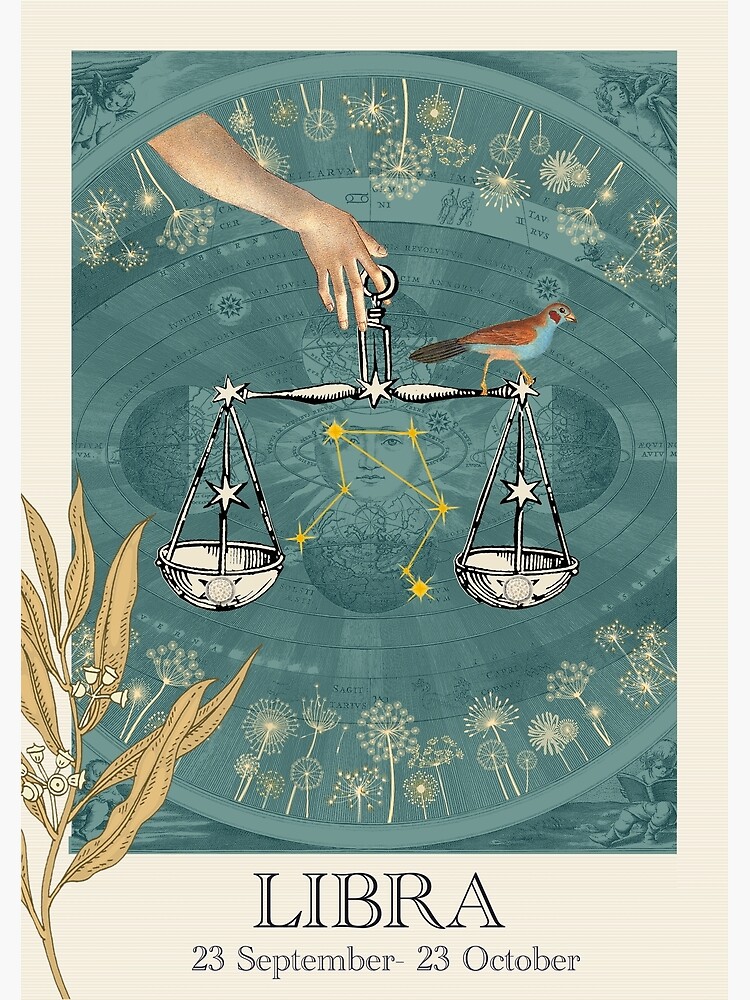This detailed illustration, presented in poster format, showcases the zodiac sign Libra with a whimsical and celestial theme. At the center of the image is a hand, drawn in a tan hue, delicately balancing a set of scales—the symbol for Libra—on its finger. The right side of the scale features a bird perched gracefully, while the left side remains empty. Surrounding the hand and scales is a cosmic backdrop filled with astrological symbols and a constellation representing Libra. A celestial face, possibly depicting the moon, adds a mystical touch to the scene.

The primary colors used in the illustration are turquoise and white, with touches of cream in the border. At the bottom of the poster, the text "Libra, 23rd September to 23rd October" prominently identifies the astrological period for Libra. The border of the image is adorned with dandelions and various flowers, and in the bottom left-hand corner, there is a yellowish-gold stem with leaves. Cherubic figures appear in the corners of the artwork, enhancing the ethereal quality of the piece.

Overall, this image is richly detailed, merging symbolic elements with artistic flair to create a captivating representation of the Libra horoscope.